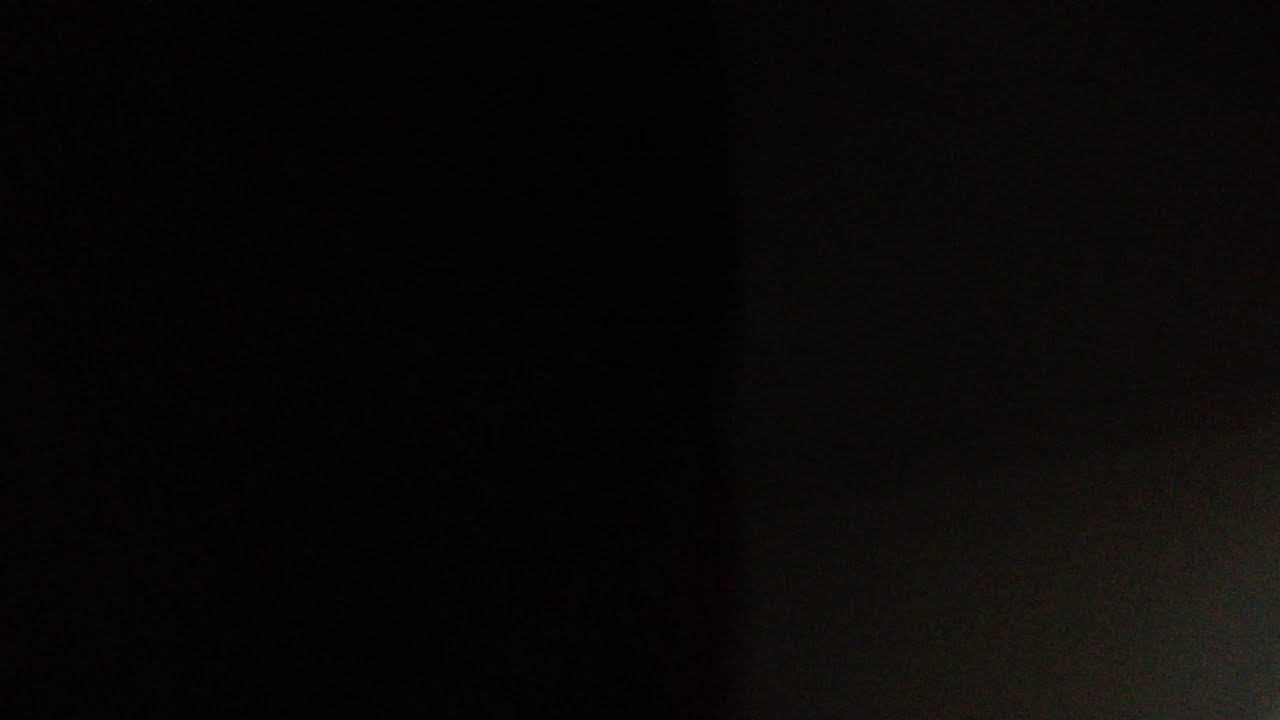The image, taken in the dark or at night, predominantly presents a smooth, untextured black background that spans across the entire frame. In stark contrast, the bottom right corner features a grainy, oval-shaped area with a mix of light colors, including green, dark green, reds, blues, and perhaps a touch of orange. This grainy region appears slightly angled, arching downwards, and gradually fading into the encompassing blackness. Despite the overall darkness, this minor section displays a faint, static-like appearance that distinguishes it from the rest of the image’s seamless black expanse.